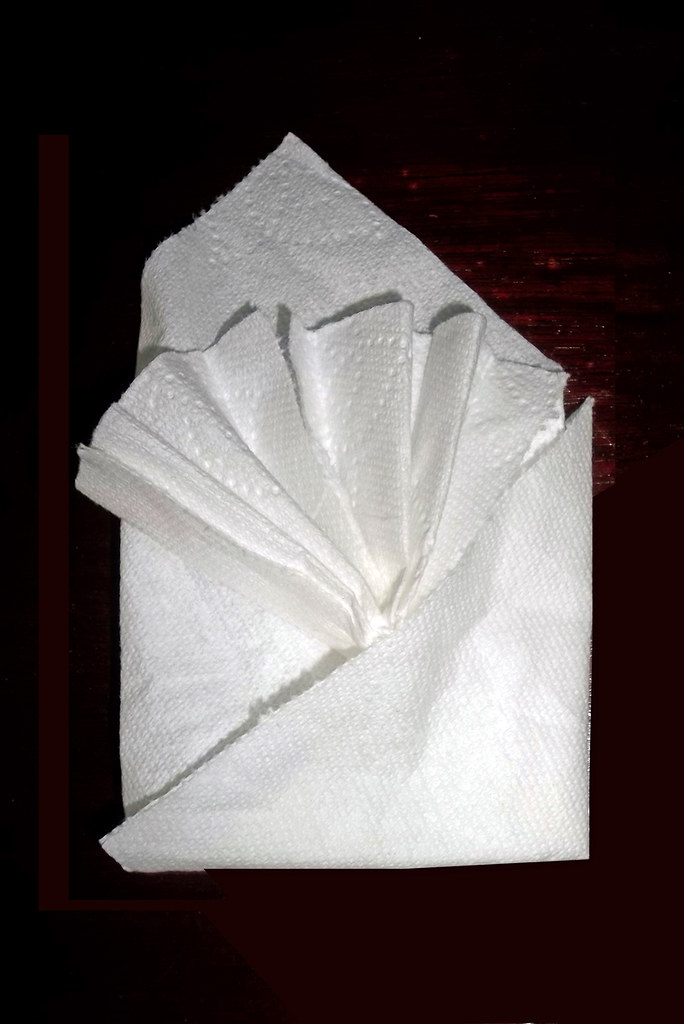This photograph captures a meticulously folded white napkin, positioned centrally against a predominantly black background accented by subtle red hues. The napkin, resembling a piece of delicate origami, features intricate textures with faint creasing at the bottom. It is folded into a square, with a triangle extending from the lower left to the upper right. From the top of this square, the napkin fans outward in a pleated, seashell-like design, illuminated by a light that highlights its creamy hue and textured surface. The background, shrouded in darkness, enhances the napkin's elegant form, giving the impression of a decorative element, perhaps part of a larger table setting.